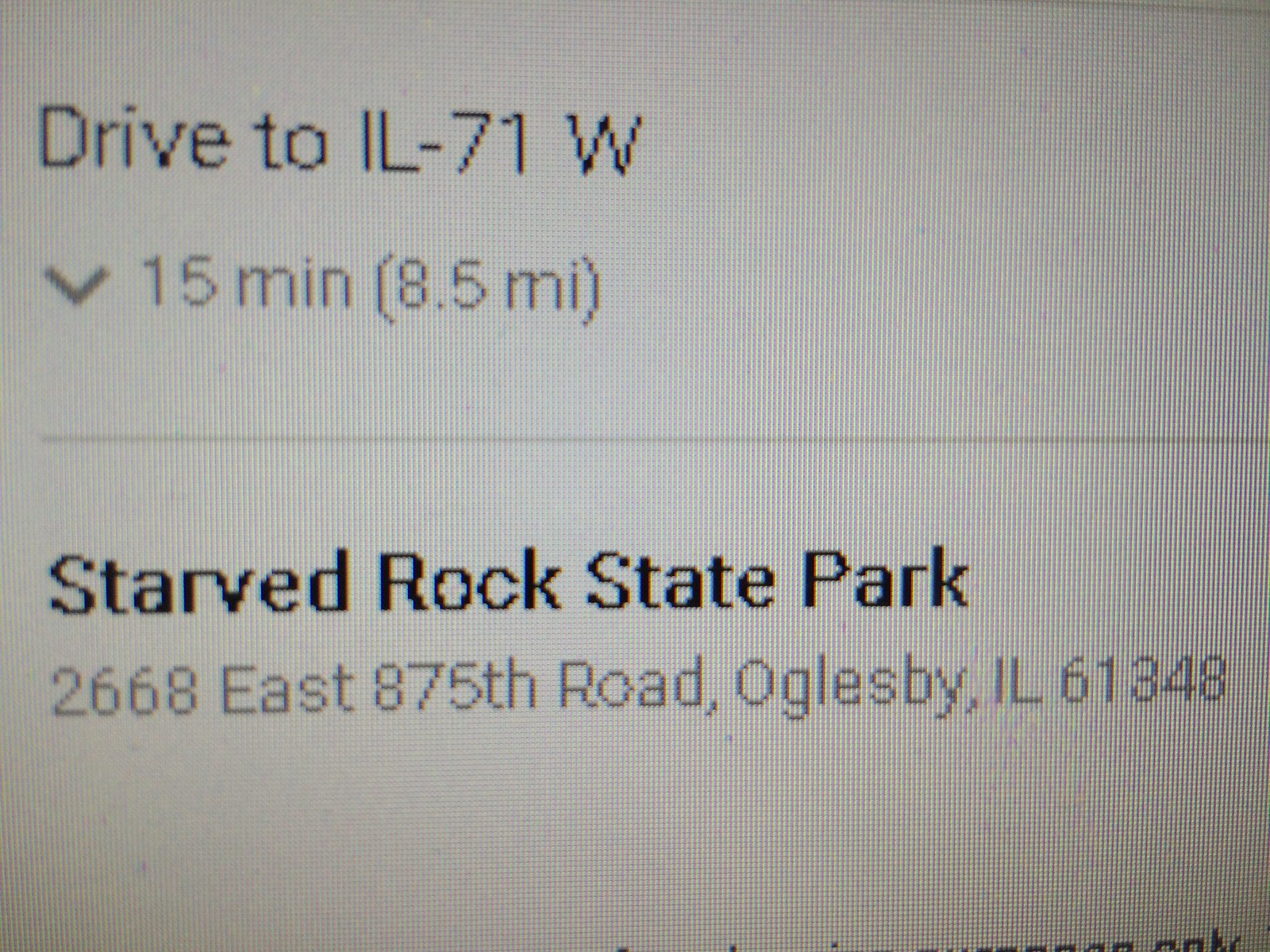This is a detailed caption for the cleaned-up photo:

"A close-up photo of a computer screen displaying map directions. At the top of the screen, the text instructs 'Drive to IL-71 West,' with an estimated travel time of '15 minutes' and a distance of '8.5 miles' indicated beneath it. To the left, there is a downward arrow suggesting the option to expand and view step-by-step directions. A small gray divider line separates this information from the content below. Towards the bottom, the destination, 'Starved Rock State Park,' along with its address, is displayed. The entire image is overlaid with faint black lines, indicative of the photo being taken directly from the computer screen, revealing the screen's pixel grid."